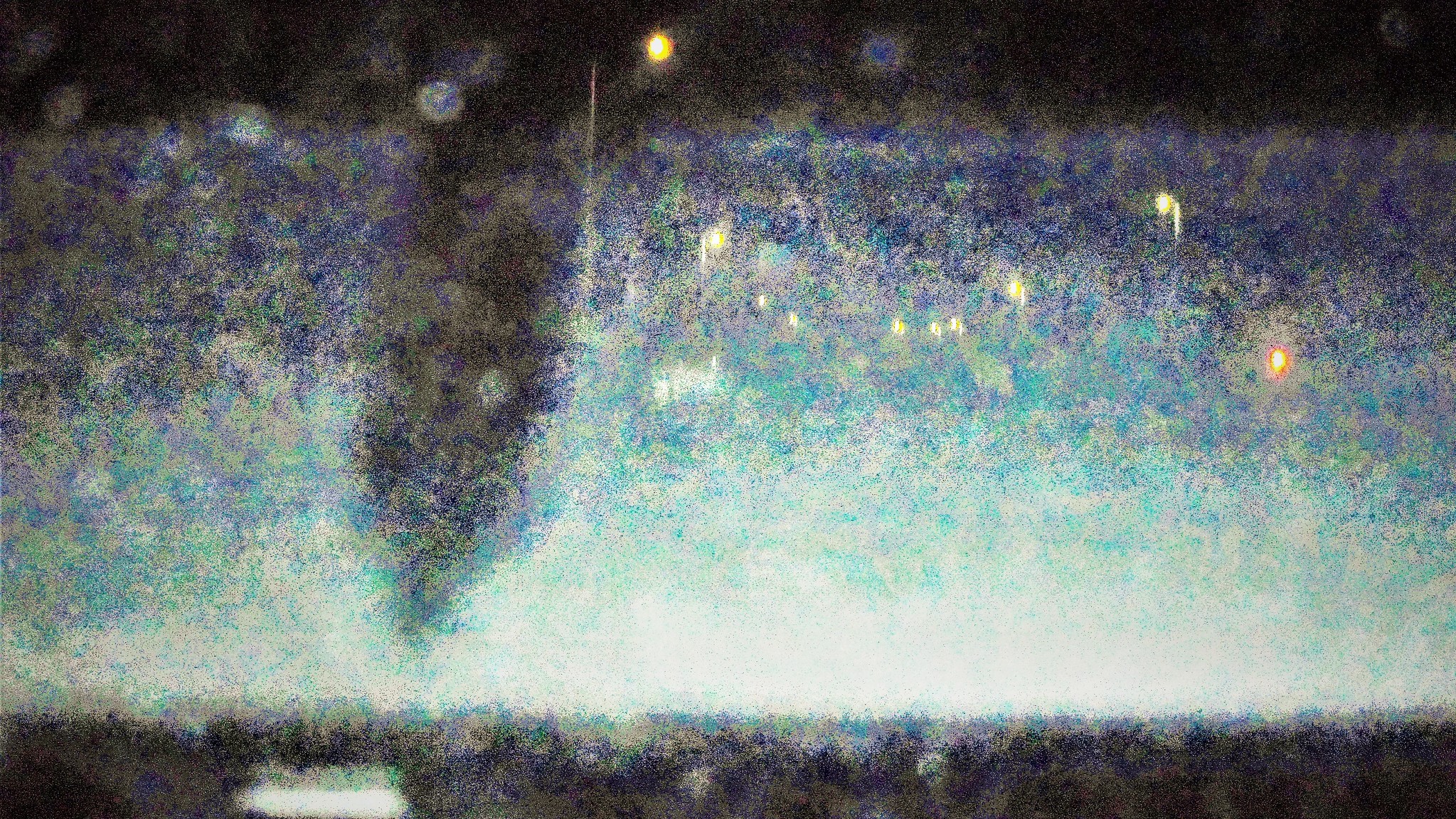This image is a colorful and highly detailed, blurry, and pixelated scene that resembles a piece of abstract artwork or a distorted photograph. The composition is structured in horizontal layers, starting with a dark black stripe at the bottom, followed by a white stripe, then a section filled with light turquoise and green dots. Further up, this transitions into a mix of blue, purple, and green dots, before culminating in another black stripe at the top. Throughout the image, there are various white, yellow, and orange dots that could be interpreted as stars, moons, or reflections, adding to the overall abstract feel. The scatter of colors and dots suggests a pointillism technique. Amidst the colorful backdrop, there appears to be a black object with a pointed tip, possibly resembling a fish diving into the colorful, water-like expanse, giving the image a vivid yet obscure quality.